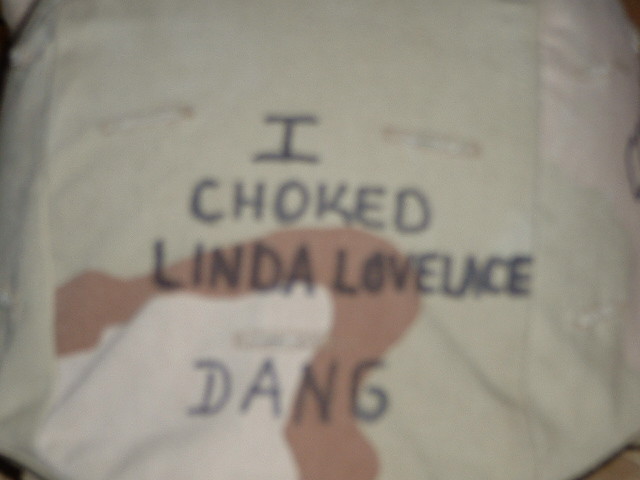This photograph features a highly out-of-focus image with a white background. Central to the composition is a piece of apparel, possibly a hat or a shirt, bearing black text. The text is stacked and reads: "I" at the top, followed by "choked" in the middle, "Linda Lovelace" beneath that, and "Dang" spelled out as D-A-N-G at the bottom. Behind the black lettering, there appears to be a red design or painting, adding depth and intrigue to the image. The overall quality of the photo seems dated, reminiscent of the 1970s or 1980s, with the focus particularly poor towards the bottom of the frame. The object, likely some sort of vintage clothing, is worn and not very clean, hinting at its age and well-loved history.